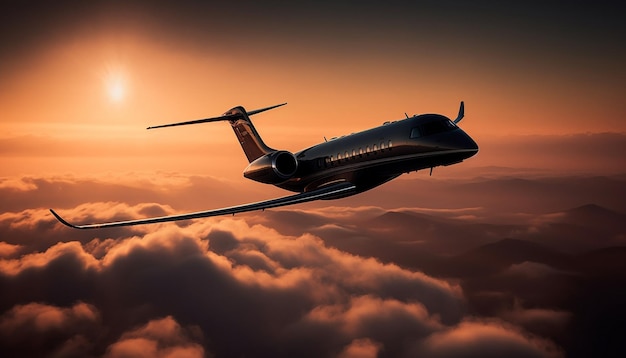In this detailed and artistic image, we see a shiny jet airplane, predominantly brown and silver, flying towards the right at an incline, suggesting it is ascending. The jet's windows are visible along the side. Beneath the plane, a sea of fluffy clouds stretches across the lower and middle left portions of the image, adding a dreamy element to the scene. The background reveals more clouds and hints at the tops of distant mountains, enhancing the overall ambiance. Towards the left, a bright, hazy area likely represents a hidden sun, casting a radiant glow across the scene, while the top of the image gradually darkens, creating a striking contrast. This interplay of light gives the entire composition a dual sense of brightness and shadow. The image has an overly aesthetic quality, resembling a highly detailed drawing rather than a traditional photograph, emphasizing its artistic nature.